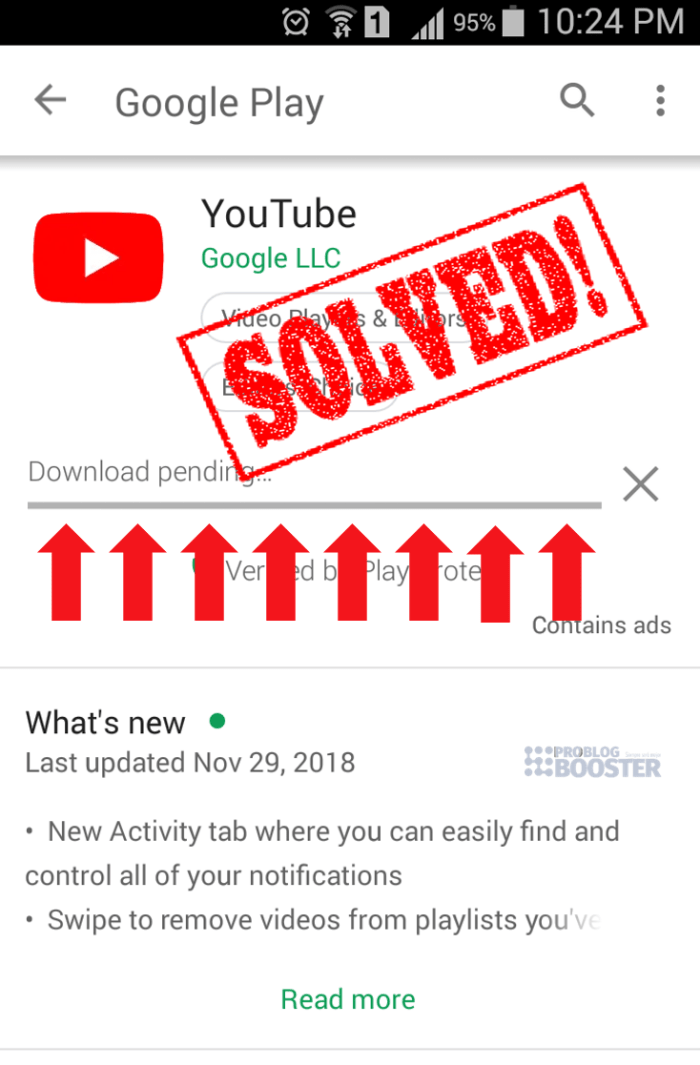The image is a rectangular screenshot of a download screen from a mobile device, set against a white background. At the top of the screenshot, a black banner displays key UI elements typical of a smartphone. From left to right, the banner shows an alarm clock icon, followed by a Wi-Fi signal indicator where three out of four lines are grayed out. Next to this is a gray rectangle with a black number "1" inside. Then, there is a connectivity symbol represented by four bars shaped like a right-angled triangle, indicating signal strength. Adjacent to the connectivity symbol, it reads "95%", followed by a battery icon, and finally, the time displayed as "10:24 PM".

Below this banner, the screenshot showcases the Google Play download screen, where an app named "YouTube by Google LLC" is currently in the "Download pending" status. Over the top half of this section, there is a prominent red stamp with the word "SOLVED" edited onto the image, drawing immediate attention.